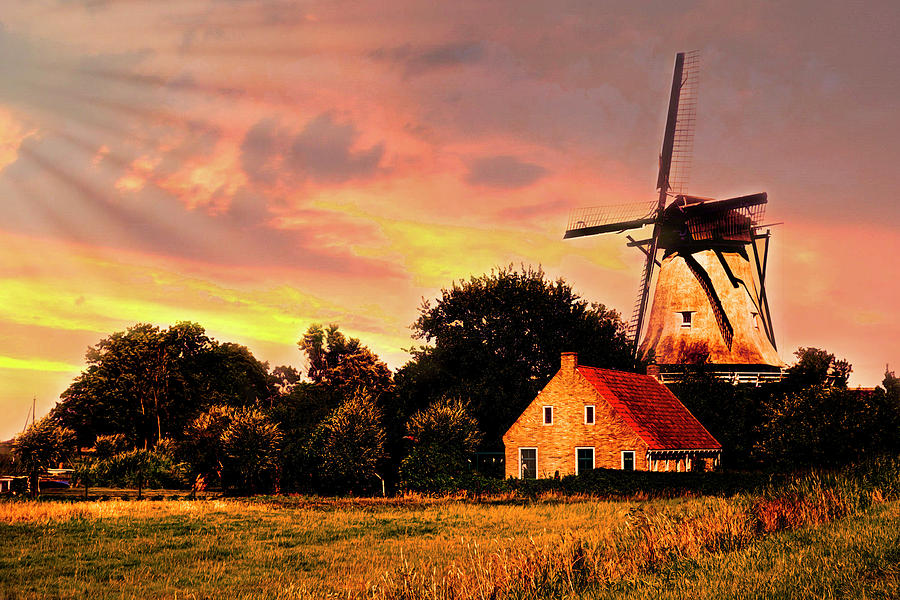This is a painting of a picturesque countryside landscape at sunset, featuring a farmhouse and a windmill. The sky is beautifully rendered with a mix of light pink, blue, gray, and yellow hues, indicating the sun is setting. The farmhouse, constructed of reddish-brown brick with white-framed windows, has a distinctive sloped red roof, likely clay tile, and two chimneys on either side. A small canopy with wooden white posts is visible on the right side of the house. Surrounding the house is a lush array of green trees, shrubs, and bushes that create a cozy atmosphere.

In front of the house, there is an expansive field of short, green grass transitioning to patches of three to four-foot-tall dried grass, possibly enclosed by a fence. Behind the house stands a four-story windmill with a dome bell-shaped body and dark brown, thin wooden propellers. The windmill, made of a reddish-brown wood, is situated behind a tree line, adding depth to the scene.

Overall, the painting exquisitely captures the serene and rustic charm of a farm area during a tranquil sunset.